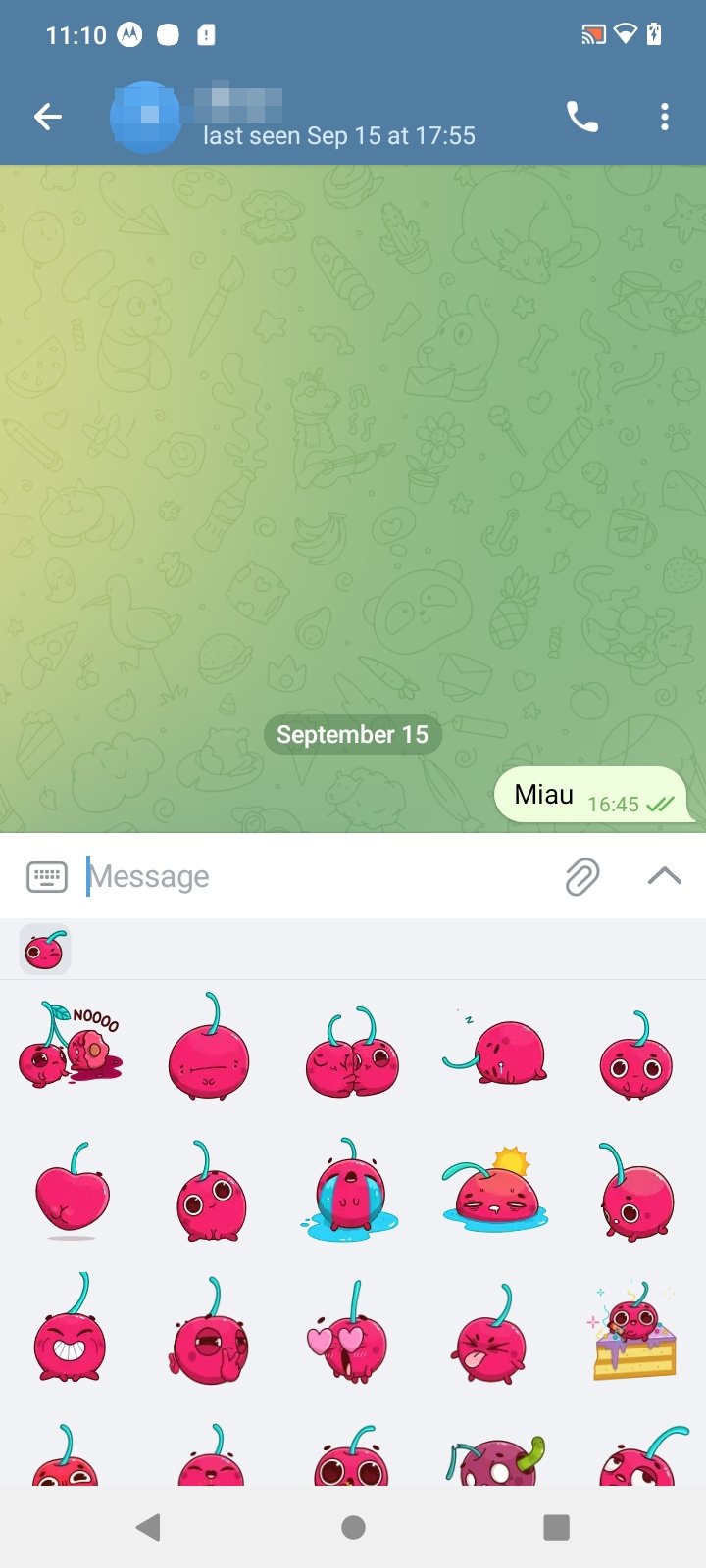A detailed image caption for the described scene would be:

"The image depicts the screen of a cell phone. At the top of the screen, the time is displayed as 11:10, accompanied by a battery icon. The interface has a blue-gray color scheme at the top, where the time, signal strength, and other icons are located. On the left of the screen, there's a left-pointing arrow, and next to it is a blue circle with the user’s name and profile icon, both of which are blurred out. Below this, the text indicates 'last seen September 15th at 17:55,' followed by a phone icon and a menu symbol composed of three vertically aligned dots.

The background wallpaper features a playful illustration of dog and panda faces, intermixed with various cartoon characters, including a dog or a lamb playing a guitar. The background colors transition from light orange-yellow to green, and the drawings are done in slightly darker shades of the same colors. Alongside these characters, there are drawings of carrots and other whimsical elements.

In the message section below, a text box appears with the letters 'M I A U' inside it, and a timestamp of '16:45.' Below that, the word 'message' is displayed, accompanied by several emoji icons. These emojis are cherries with red bodies, green stems, and small triangles meant to represent eyes in a darker red shade."